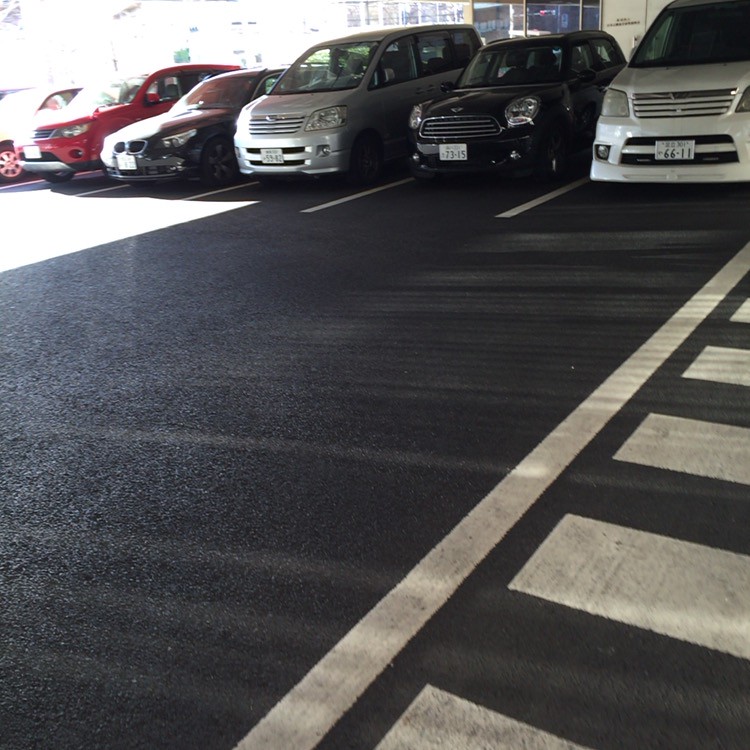This photograph captures a lineup of six cars parked side by side in what appears to be a parking garage or parking lot with a dark gray asphalt surface. Along the right bottom corner of the image, a distinctive crosswalk with white horizontal and thick vertical lines enhances the scene. The cars, varying in style and color, span from a white vehicle at the far left—partially cut off in the photo—through a sequence of a black Mini Cooper, a silver-colored minivan, a black coupe, a red SUV, and an unidentified vehicle largely obscured by intense sunlight. Each car is notable for its front license plate featuring two numbers followed by another set of two numbers. The setting denotes a transition space, potentially linking different buildings such as an airplane terminal or hotel, and features shadows suggesting covered parking. The vehicles are parked in front of a business-front lined with windows, situating the scene in a busy, functional outdoor environment.